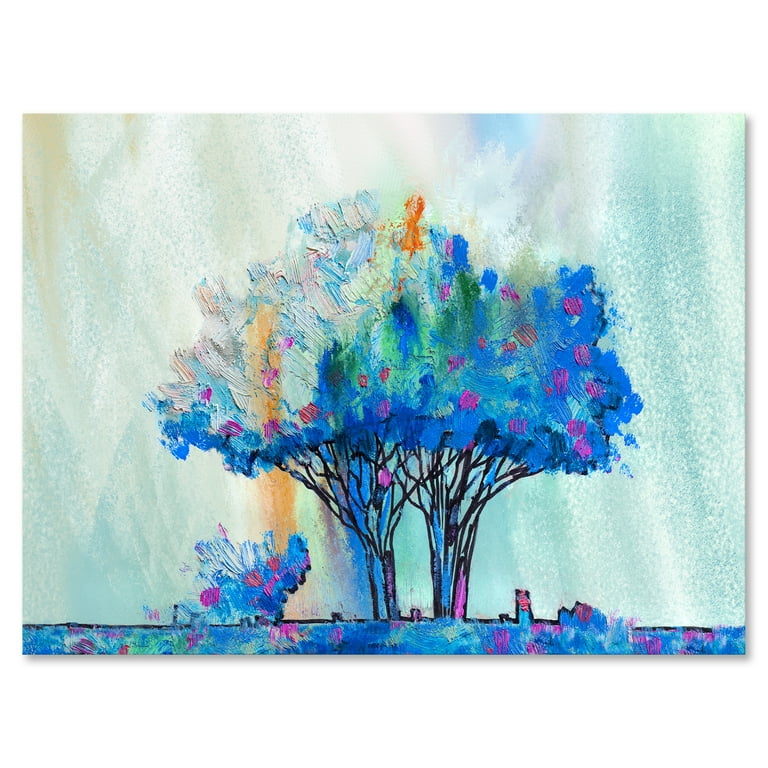This image depicts a semi-abstract watercolor painting centered around two interconnected trees. The trunks of the trees stand side by side, with branches weaving together to form a larger, unified canopy. The foliage is a rich blend of blues, reds, greens, purples, and oranges, creating a vibrant contrast against the lighter, streaky sky painted in pale blues, whites, and hints of orange. Below the trees, the ground is represented in various blue tones with splashes of additional colors, suggesting depth and distance with hints of a far-off cityscape. A larger bush sits to the left of the trees, while a smaller one is to the right, mimicking the tree's colorful palette. The brushwork combines both watercolor fluidity and acrylic-like textures, adding dimension to the leaves and sky, making the trees and the landscape the most striking elements of this intricate and colorful artwork.